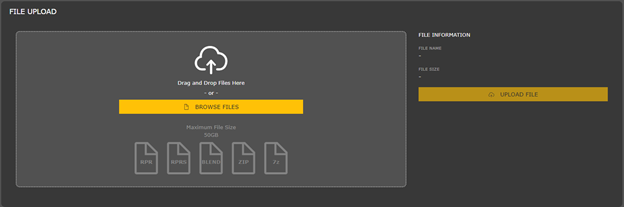**Detailed Descriptive Caption:**

The image features a predominantly black background with a dark gray rectangular section on the left side. At the very top center, the text "FILE UPLOAD" is prominently displayed in all capital letters and in white. Inside the dark gray rectangle, there is an icon of a cloud with an upward-pointing arrow, symbolizing file upload functionality. Below this icon, the text "Drag and drop files here" is placed, guiding users on how to upload files. Beneath this instruction, there's an orange rectangle with the text "Browse files," indicating an alternative method for selecting files. Below the orange button, a note states "Maximum file size: 50 gigabytes."

Directly under this note are several icons representing different file formats, notably displayed as pieces of paper with the top right corners folded down. From left to right, the icons are labeled: "RPR," "RPRS," "Blend," "Zip," and "7Z." On the right side of the image, aligning vertically, there is a section titled "File Information," listing "File Name" and "File Size" fields. Further down, another dark orange rectangle with the text "Upload File" is positioned, meant to finalize the file upload process.

The image is clearly designed with functionality in mind, offering no elements related to people, animals, plants, vehicles, or any photographic content. Its horizontal orientation and structured layout suggest it is a user interface design for a file uploading feature.